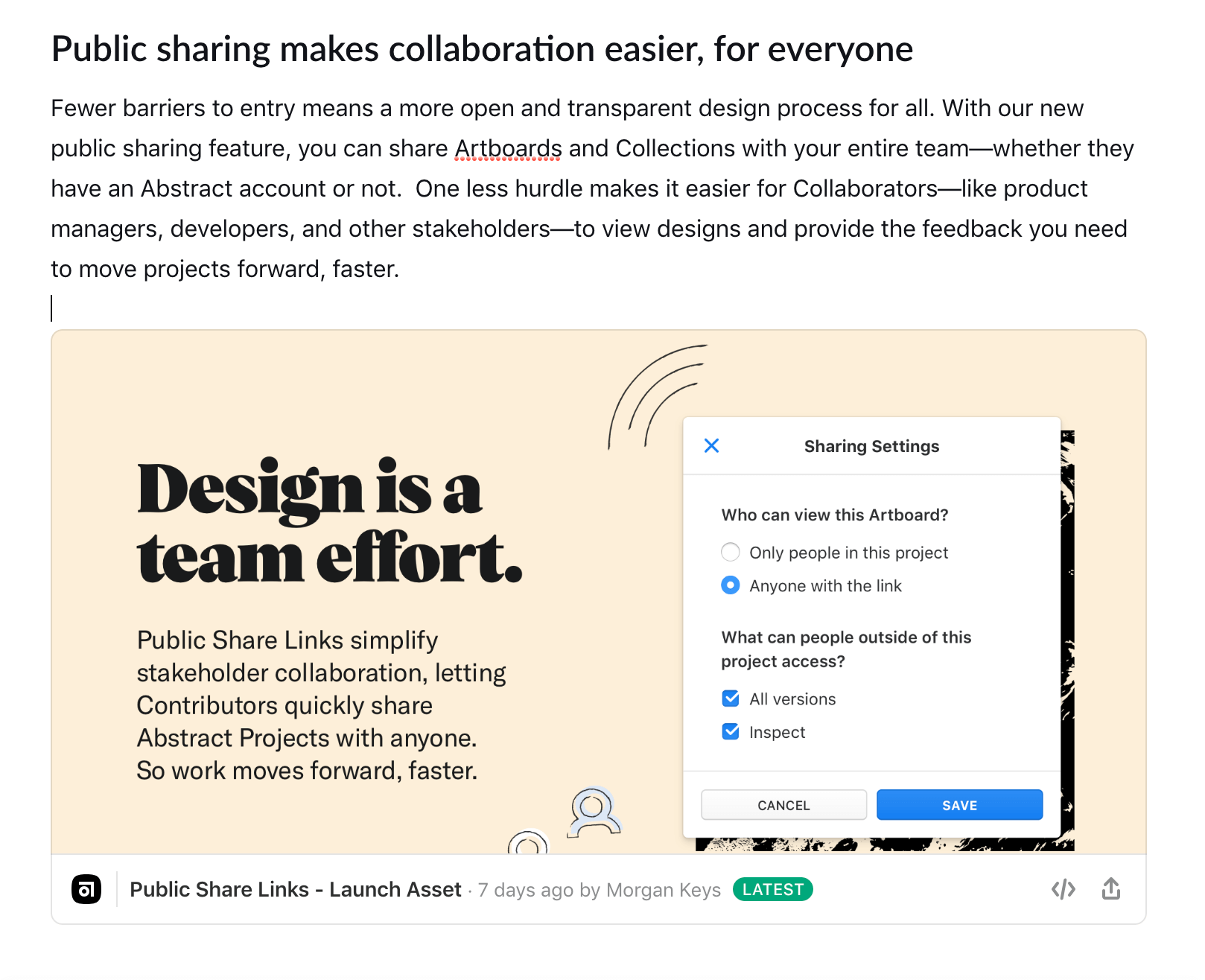The image is a left-to-right horizontal screenshot, likely captured from a smartphone, potentially an Android or an iPhone. The background transitions subtly between a beige hue and white, indicating it was captured from a computer screen with those colors as the backdrop.

At the top, bold black text declares, "Public sharing makes collaboration easier for everyone." Below this headline, a secondary line of text articulates, "Fewer barriers to entry mean a more open and transparent design process for all. With our new public sharing feature, you can share artboards and collections with your entire team whether they have an abstract account or not. One less hurdle makes it easier for collaborators like project managers, developers, and other stakeholders to view designs and to provide feedback, the feedback you need to move projects forward faster."

In the section set against the peachy, beige background, the text states, "Design as a team effort," followed by a brief explanatory blurb. It also features a white inset box titled "Shared settings." Below this title, options allow users to specify "Who can view this artboard," either "Only people in this project," or, as selected, "Anyone with this link." Further settings enable users to determine "What people outside of the project can access," with "All versions" and "Inspect" selected. Two buttons labeled "Cancel" and "Save" sit at the bottom of this box. Finally, at the very bottom of the image is the text, "Public share links, launch asset."